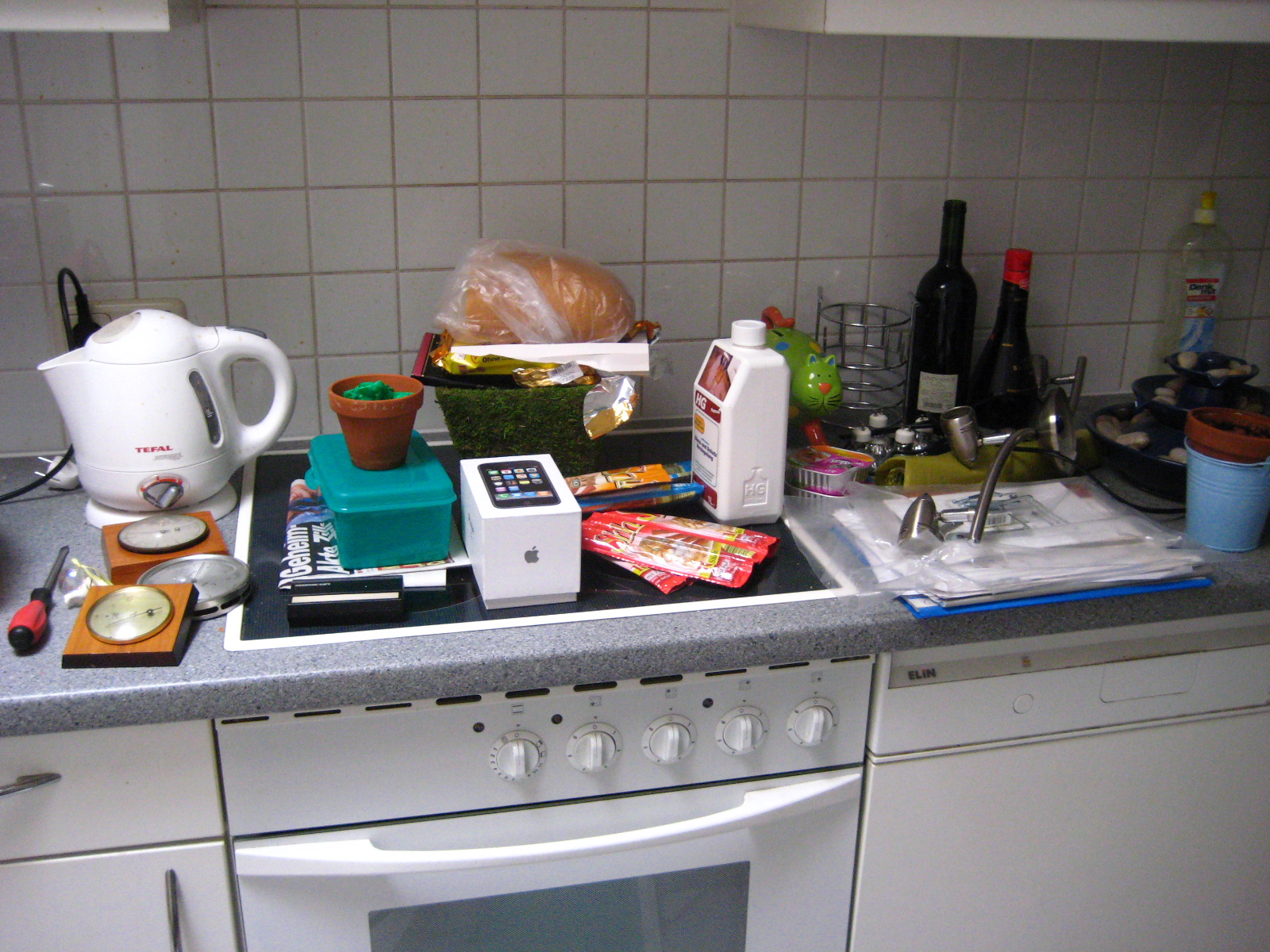This photograph captures a section of a highly cluttered kitchen characterized by its various appliances and objects scattered across the countertop. 

The backsplash is composed of square white tiles with beige grout, contributing to an overall simplistic and average design. The countertop itself is a gray speckled Formica that extends across the visible area. 

To the right, there is a series of kitchen appliances starting with a white dishwasher that has a gray strip at the top, followed by a standard white oven. Adjacent to the oven is a black flat-surface cooktop. Beside the cooktop, there is a kitchen cabinet with a drawer, both of which feature gray handles.

The countertop, which appears to also extend over the cooktop, is cluttered with a variety of items arranged from left to right. These include an electric tea kettle, a coffee maker, a red and black screwdriver, and two flat brown clocks made of wood with gold accents. There is an aqua-colored plastic container, a terracotta pot containing a green plant, a basket filled with bread, a white box holding an iPhone, several red pieces of paper, a white plastic bottle, and some scattered papers. Additionally, there are bottles in the background, one of which appears to be a wine bottle.